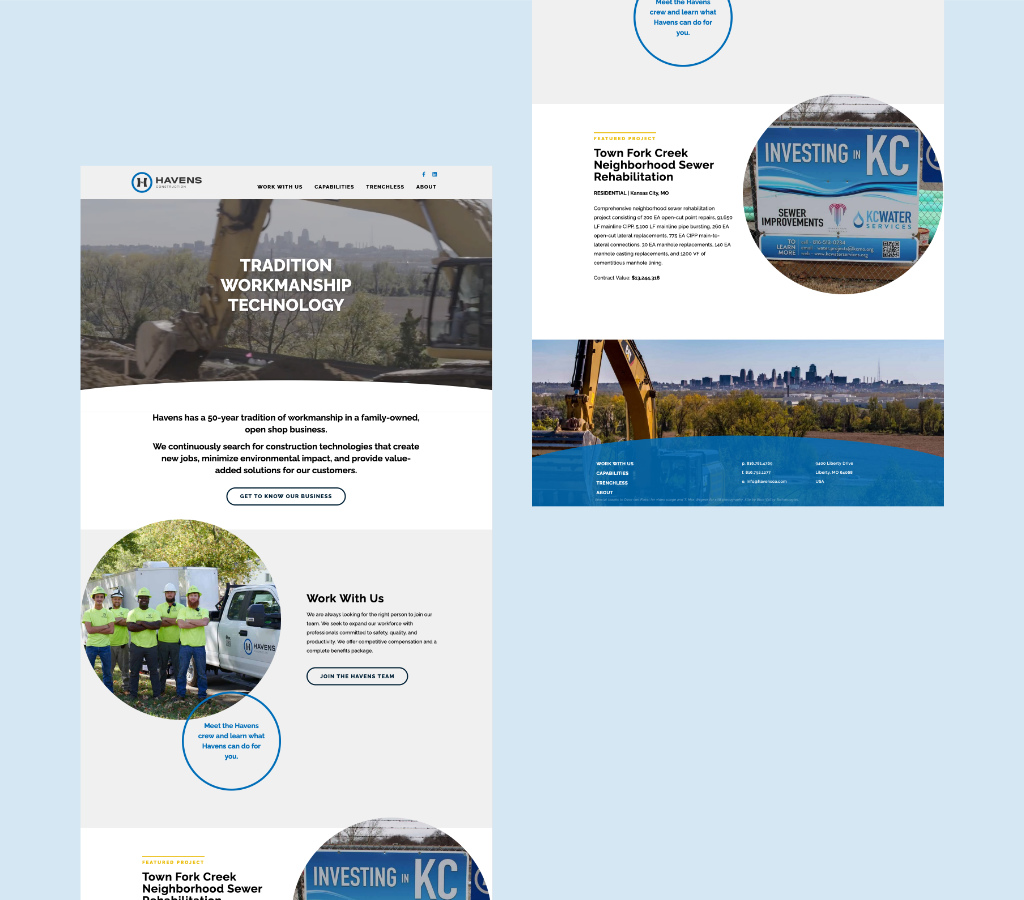This image showcases a website laid out in two distinct sections, with the top half displayed on the left and the bottom half on the right. The backdrop of the webpage features a serene sky blue, while the main content is presented on a canvas of white and tan hues. 

In the upper section, key navigation headers such as "Havens", "Work with Us", "Capabilities", "Technologies", and "About" are prominently displayed. Below these, the text highlights Havens' legacy with a statement: "Tradition, workmanship, technology. Havens has a 50-year tradition of workmanship in a family-owned open shop business. We continuously search for construction technologies that create new jobs, minimize environmental impact, and provide value-added solutions to our customers."

Encouraging engagement, it continues with a prompt: "Get to know our business. Work with us, join the Havens team, meet the Havens crew, and learn what Havens can do for you." 

An image accompanies this section, depicting a white truck branded with "Havens" and five individuals clad in neon green shirts and hard hats standing beside it, symbolizing the workforce and teamwork ethos.

On the right side, representing the lower part of the webpage, the focus shifts to a project named "Town Fork Creek Neighborhood Sewer Rehabilitation." A sign within the image reads: "Investing in KC, sewer improvements, KC Water Services to learn more," supplemented by a QR code for additional information. This section is visually supported by images of various construction vehicles, trucks, and scenic views of tree lines and distant cityscapes, illustrating the project's environmental context and urban integration.